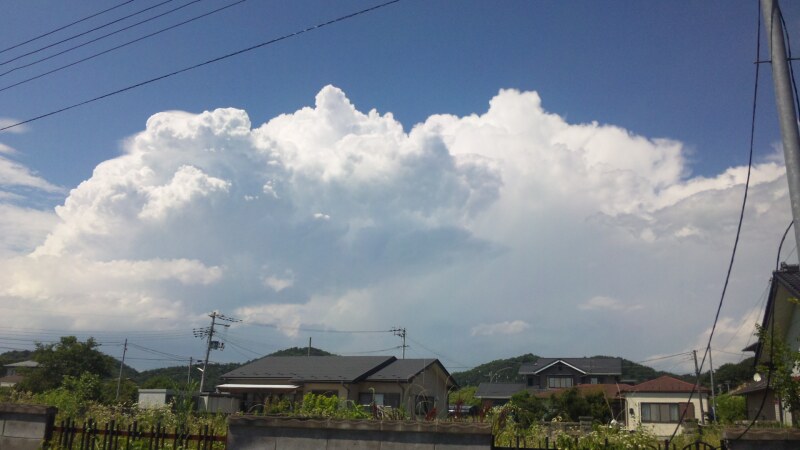This photograph captures a picturesque neighborhood set against a backdrop of rolling hills or mountains in the far distance. The homes, mostly brown with black roofs, stand out, with one notable tan house featuring a red roof. Trees and bushes, some adorned with white or red flowers, dot the landscape and envelop the properties, creating a lush environment. In the foreground, a stone and iron fence can be seen, adding to the charming residential setting. Looming large in the sky are thick, fluffy white clouds, contrasting with the clear, blue expanse and accentuating the peaceful atmosphere. Telephone poles with wires strung between them traverse the scene, anchoring it in a serene blend of nature and suburban life.